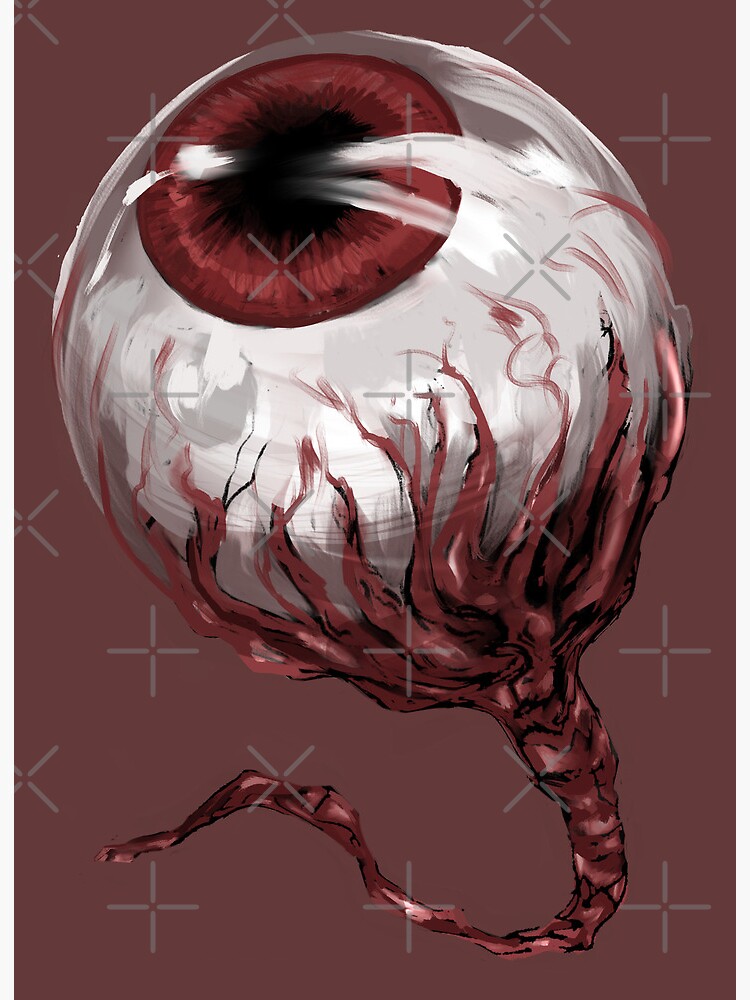This digital artwork depicts a large, detached eyeball set against a maroon, brick-red background. The eyeball, prominently featured in the center, has a vivid red iris with subtle white highlights and black shading. The sclera, or the white part of the eye, contrasts starkly with the red veins that snake across its surface and connect to a meaty tendril. This tendril extends from the back of the eye, tapering off into a thin, hook-like shape that curves to the left. The pupil gazes upwards towards the 11 o'clock position, giving the piece a surreal and slightly eerie aura. The image also includes scattered white T's and X's across the background, adding to the sci-fi and futuristic feel of the composition. The intricate details of the eye, along with the cohesive red hues, create a striking and memorable visual impact.